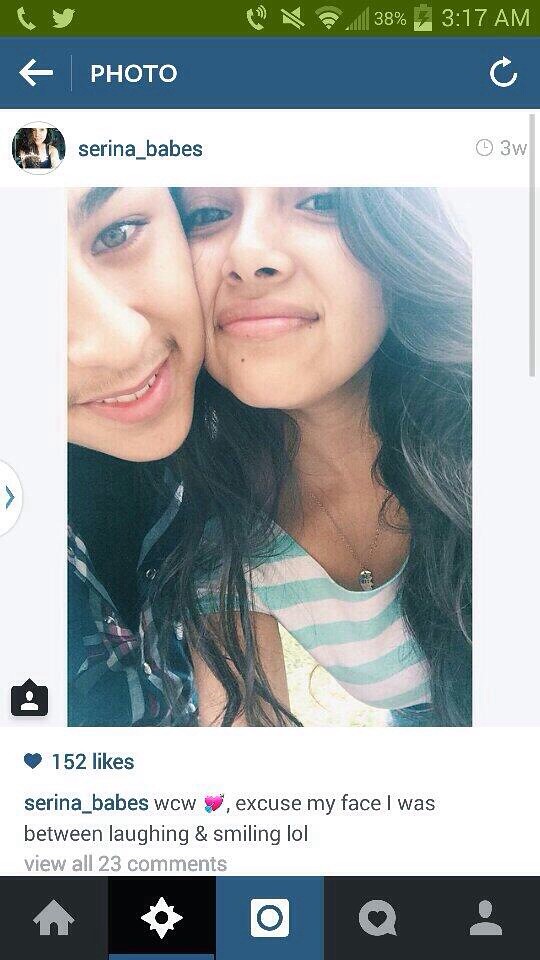Here's a cleaned-up and detailed caption combining information from all three sources:

---

The screenshot shows a Facebook post viewed on a mobile phone. At the top, there's a green status bar with icons indicating phone signal, Twitter notifications, battery life at 38%, and the time, 3:17 AM. Below it, the app interface features a blue banner with a left-pointing arrow and the word "Photo" on the left, and a refresh icon on the right.

The main content displays a post by Serena Babes, evidenced by a small circular profile picture of a young woman with long, dark hair, to the left of the username "Serena_Babes." To the right, a clock icon indicates the post was made 3 weeks ago. 

The photo itself captures a young woman cheek-to-cheek with a young man, who is partially off-screen. Both have light brown skin and dark hair. She wears a blue and white t-shirt and a necklace. Only the lower part of her face is visible, while the young man’s face is cut off on the left side.

Below the image, a blue heart icon indicates the post has received 152 likes. Serena's caption reads: "WCW ❤️ Excuse my face, I was between laughing and smiling lol." It's followed by a prompt to "View all 23 comments." At the bottom of the screen, there are icons for home, star, camera, a heart with a comment bubble, and a people button.

---

This provides a comprehensive description by emphasizing repeated and shared details across all sources.